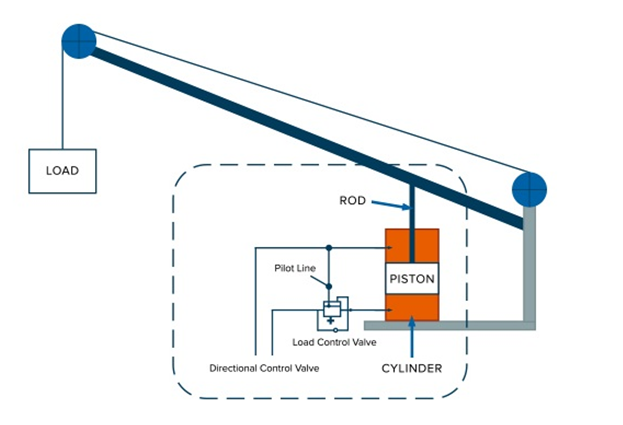This digital diagram depicts an intricate crane or pulley system with detailed labeling and a simplistic color scheme. The crane features a gray L-shaped mounting plate on the right, extending an arm towards the top left and supporting two pulleys. An orange piston housed inside a white cylinder is clearly visible, connected to a blue rod. This rod extends to the top left and ends near the second pulley, holding a load. The load is suspended from a line that runs from the first pulley on the mounting plate to the second pulley, forming a functional lift mechanism. Central to the operation are the detailed hydraulic components: a pilot line, a load control valve, and a directional control valve within a dashed square across the diagram. The diagram uses strategic colors—white, black, blue, gray, and orange—to differentiate the various elements, showcasing the mechanical interplay that allows the crane to lift and lower the load effectively.